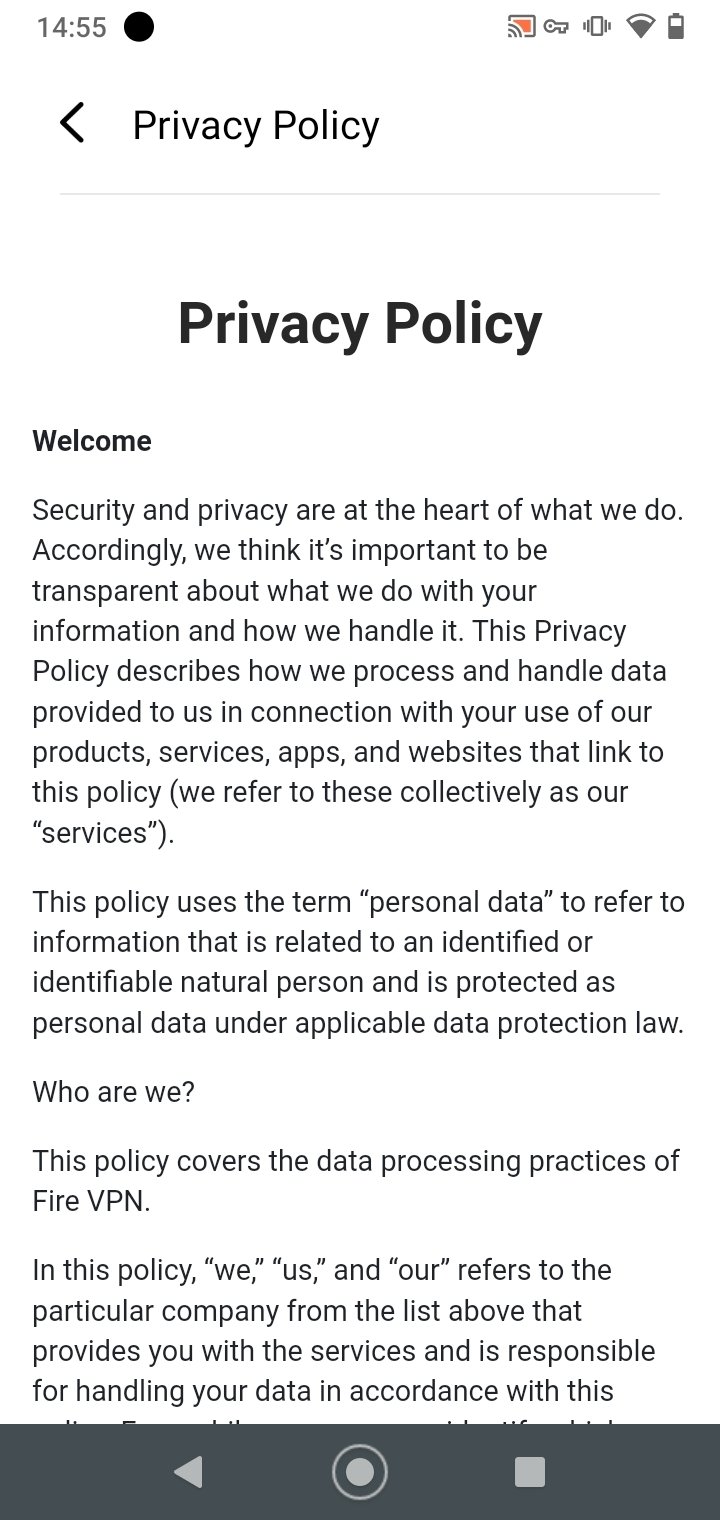The screenshot captures an email displayed on a phone with a white background. The phone status bar at the top shows the time as 14:55, with indicators for battery, Wi-Fi, and signal strength on the right side. Beneath the status bar, the title "Privacy Policy" is prominently displayed in large black letters, accompanied by a left-pointing arrow.

The email body is set against a white backdrop with black text and begins with a welcoming message, emphasizing the importance of security and transparency in handling user information. It states: 

"Welcome, security and privacy are at the heart of what we do. Accordingly, we think it's important to be transparent about what we do with your information and how we handle it."

The document proceeds to outline its purpose, explaining that the privacy policy details the methods of processing and handling data provided during the use of their products, services, apps, and websites linked to this policy. The term "personal data" is defined as information related to an identified or identifiable natural person, protected under applicable data protection law.

An introductory section labeled "Who are we?" clarifies that the policy pertains to FHIR VPN, mentioning that terms like "we," "us," and "our" refer to the specific company branch providing the services and responsible for data handling in accordance with the policy.